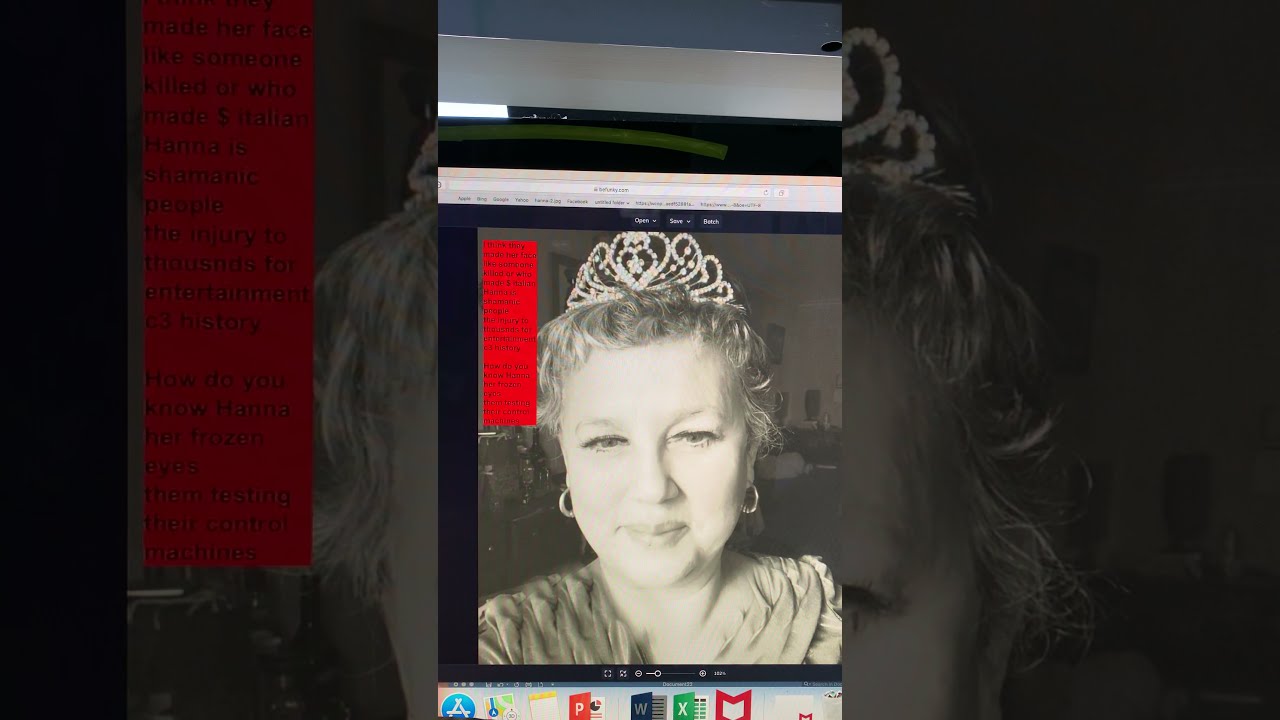The image features a centered computer screen displaying a black and white photograph of a woman adorned with a jewel-encrusted tiara. The woman has her slightly curly hair pulled back and up, showcasing her ring-shaped earrings. Her expression is a small, closed-mouth smile as she looks slightly downward or straight ahead. On the upper left corner of the screen, there is a faded red box containing illegible black text. The screen shows typical Mac widgets at the bottom, including icons for applications like Word, Excel, and the App Store, along with other colored widgets that add accents of blue, white, red, and green. The image appears to be either a screenshot or a photograph taken of a computer monitor, capturing the combined display of a faded, grayscale portrait and the surrounding digital interface.